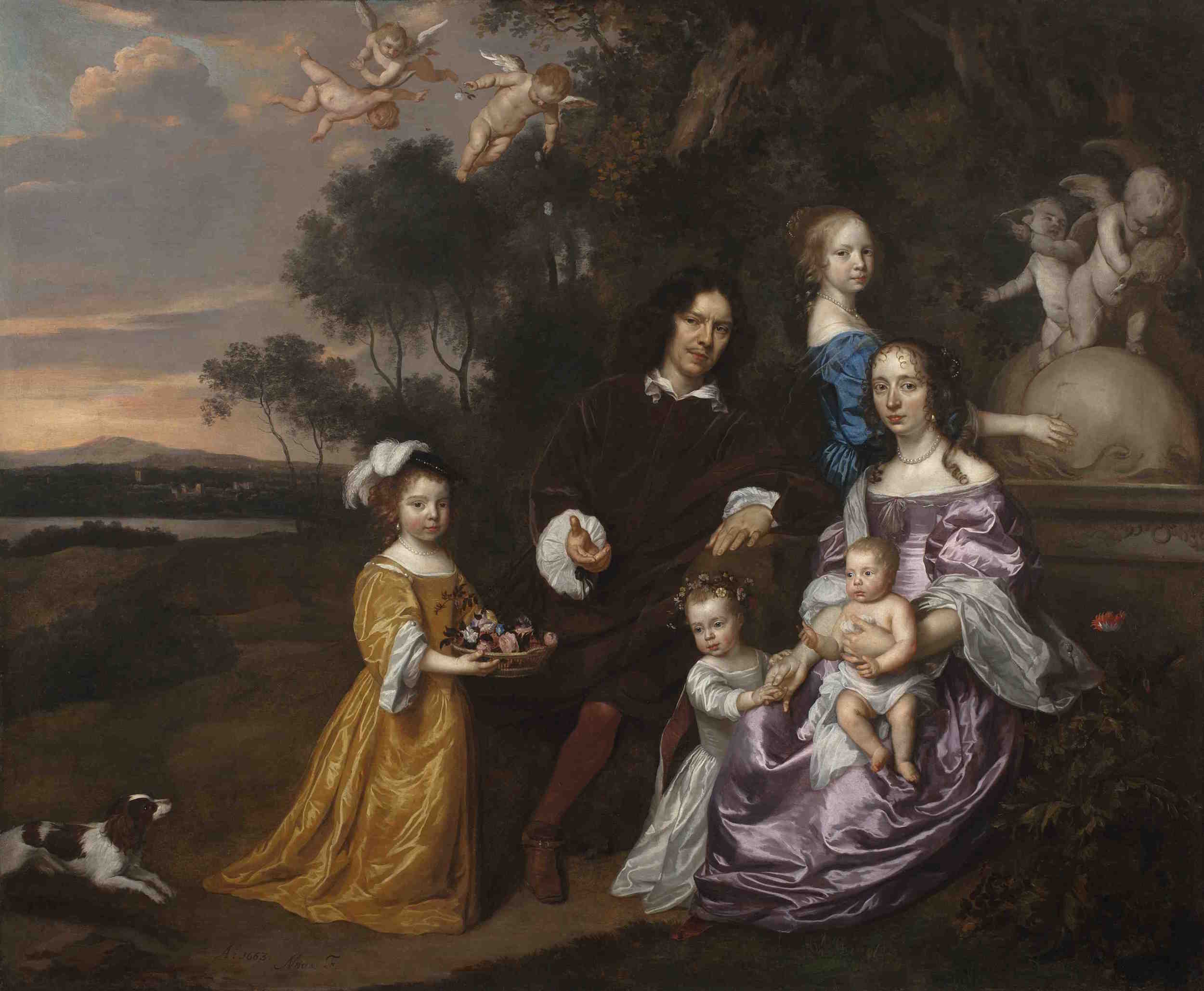An outdoor Renaissance-style painting depicts a serene family scene with rich details and vibrant attire. At the center sits a man with long, curly dark hair, dressed in a dark maroon gown with white sleeves and tall brown boots. Beside him, a woman in a flowing purple gown holds a baby wrapped in a white cloth, with a neutral expression on her face. The family includes various children; to the left, a young girl with curly red hair and a white feather headdress wears a long-sleeved gold gown that drags on the ground. She holds a basket of flowers and is accompanied by a brown and white spaniel, gazing up at her. Another child stands behind the woman in a blue gown, likely a teenager, and a small toddler stands by the mother's side. 

Descending from the partly cloudy, early evening sky with its pink, gray, and blue hues are angelic babies with white wings. A sculpture of an angel is positioned to the right. In the background on the left, there are rolling hills, patches of green grass, and a serene lake under the partly cloudy sky. The setting includes gray clouds with glimpses of blue, creating a calm yet dramatic atmosphere. The image beautifully merges the natural outdoor setting with elements of divine and familial tenderness, encapsulating the elegance and detail typical of Renaissance artwork.